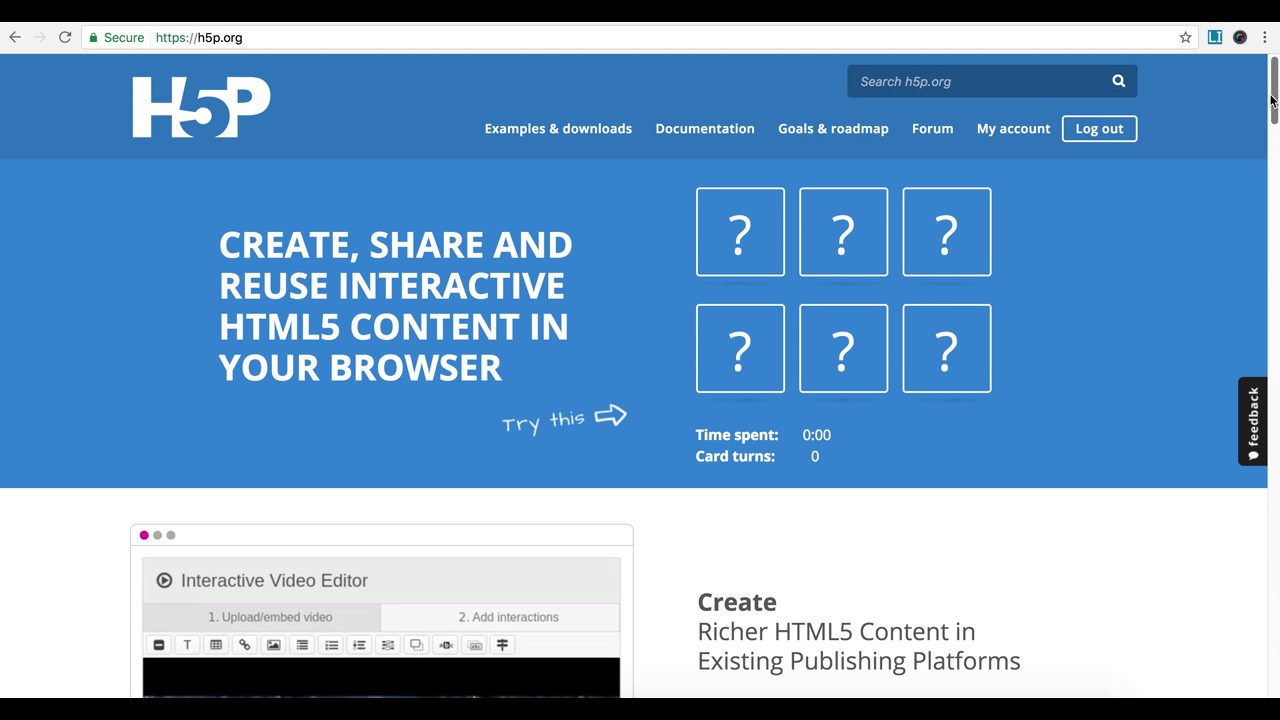Here is a cleaned-up version of the caption for the image of the H5P website:

---

This is a screenshot of the H5P website, featuring a dark blue header with the company's logo positioned on the top-left corner. Next to the logo is a menu bar that includes the following options: Examples and Downloads, Documentation, Goals and Roadmap, My Account, and a Logout button located on the far right. Above the Logout button, there is a search bar. The main body of the webpage has a lighter blue background, adorned with white, all-caps text that reads: "CREATE, SHARE AND REUSE INTERACTIVE HTML5 CONTENT IN YOUR BROWSER." To the right of this text, there are six boxes arranged in two rows of three, each containing a question mark. Below these boxes, text reads: "Time Spent: 0, Cards Turned: 0," along with a prompt that says "Try this" accompanied by an arrow pointing at the boxes. The section below this shifts to a white background, showcasing an image of a browser on the left side depicting an interactive video editor with tabs labeled "Upload and Embed Video" and "Add Interactions." On the right side, text reads: "Create richer HTML5 content in existing publishing platforms."

---

This descriptive caption gives a clear and detailed overview of the webpage's layout, design elements, and text content.